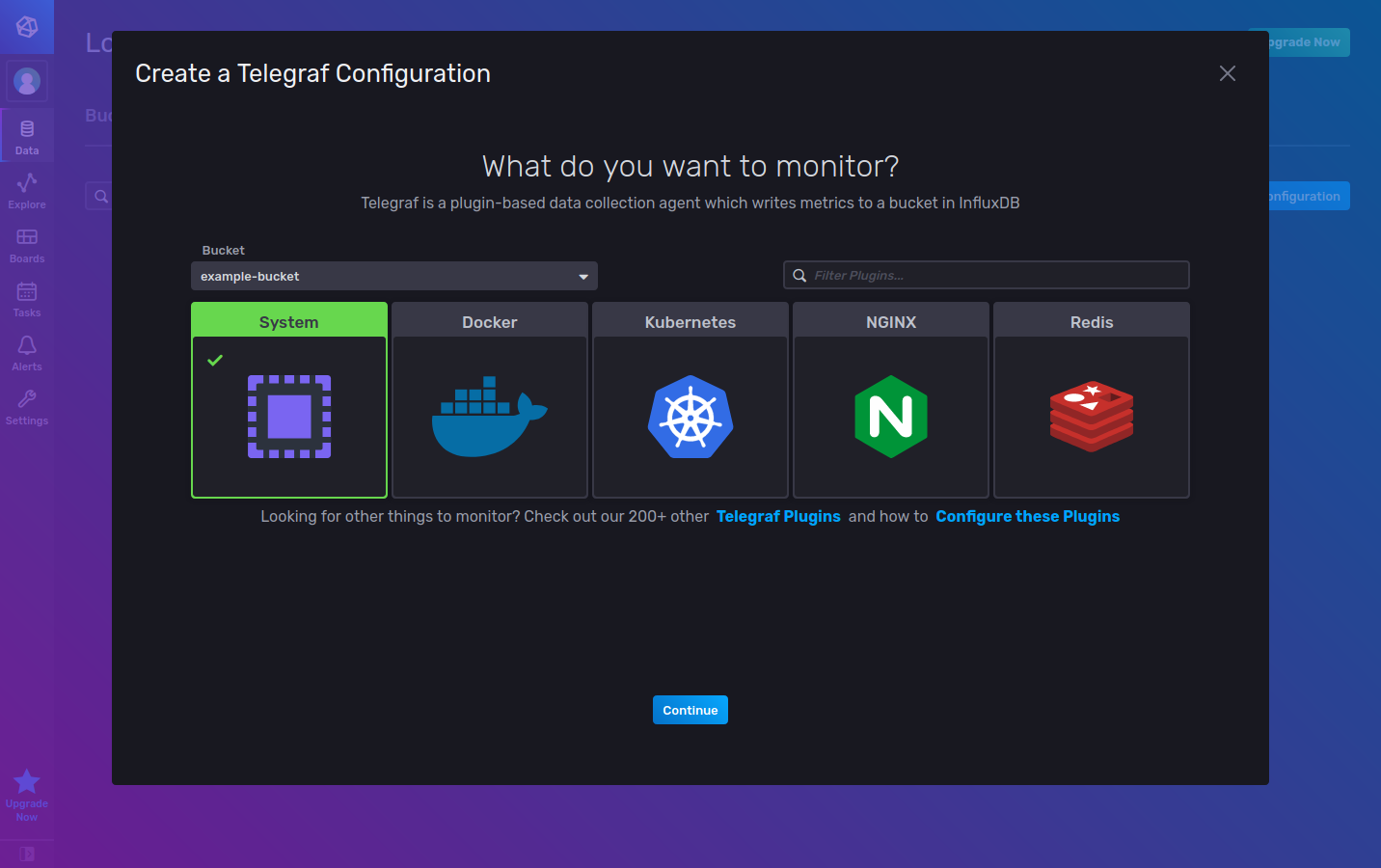This image is a screenshot of a webpage with visually striking background colors, transitioning from shades of purple on the left to shades of royal blue on the right. However, this beautiful backdrop is largely obscured by a prominent, rectangular pop-up box that dominates the center of the screen, allowing only glimpses of the background along the edges and slightly at the top and bottom.

The pop-up box itself has a sleek black background. In the upper left corner, in white font, it reads "Create a Telegraf Configuration," with "Telegraf" spelled out as T-E-L-E-G-R-A-F. Centrally displayed in larger white font is the question, "What do you want to monitor?" Beneath this, in smaller white text, is an explanation: "Telegraf is a plugin-based data collection agent, which writes metrics to its bucket in InfluxDB."

Below this text, there are icons representing five different programs, arranged horizontally from left to right. Each icon is accompanied by the program name at the top:

1. **System**: This is the selected option, indicated by a green check mark and a green-topped box. Its icon is a purple square within a black square, bordered by a purple dotted outline.
2. **Docker**: Featuring a stylized, blue whale drawing.
3. **Kubernetes**: Resembling a ship's steering wheel, symbolic of maritime navigation.
4. **NGINX**: Depicted as a green hexagon with a white letter "N" at the center.
5. **Redis**: Illustrated as a 3D stack of three red layers forming a cube shape, topped by small geometric shapes—a star, a circle, and a triangle.

The pop-up effectively focuses the viewer's attention on the task of setting up monitoring criteria while giving a subtle hint of the webpage's colorful layout remaining in the background.